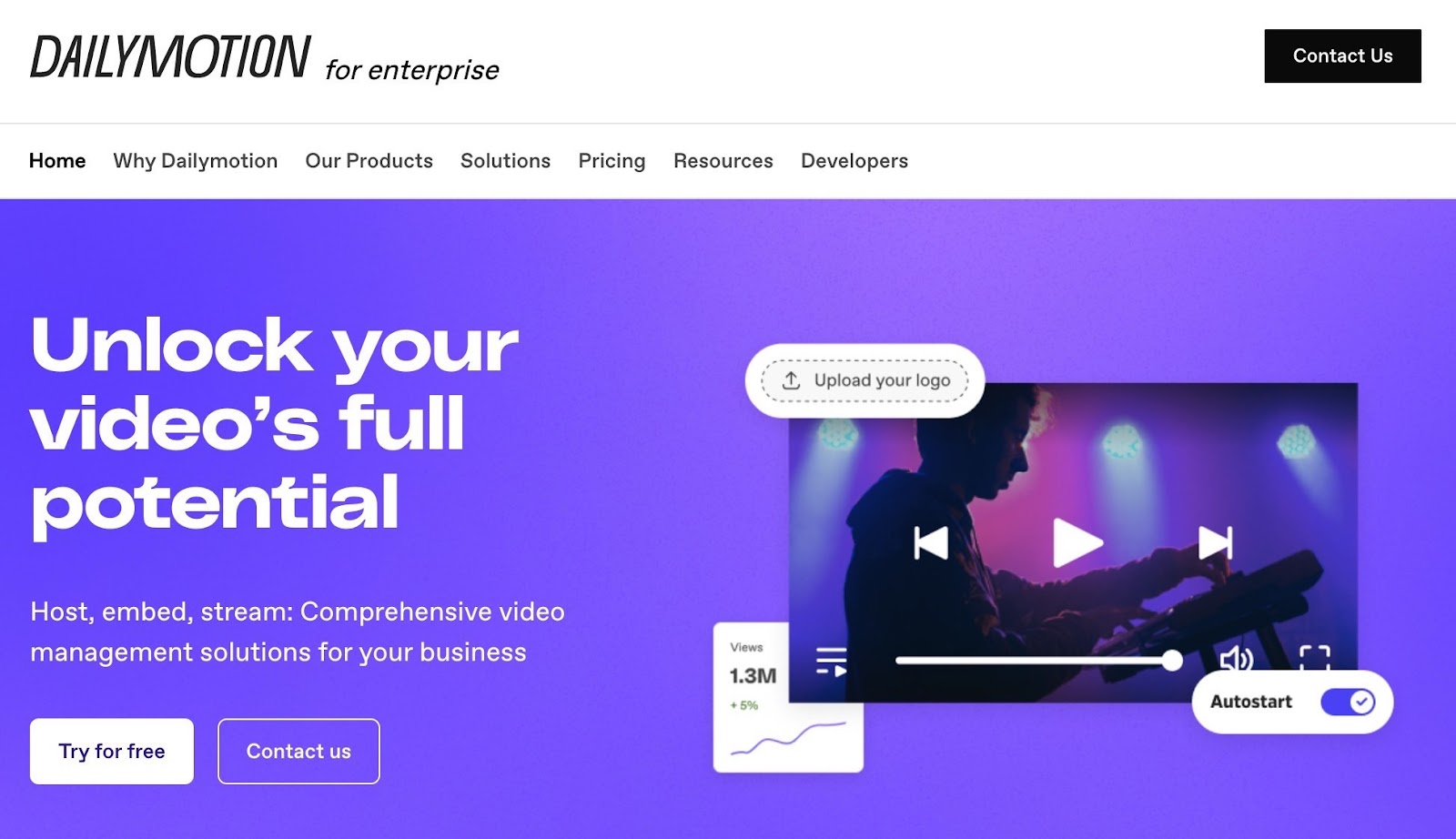The image is a screenshot of a business-focused website, designed for enterprises to harness the power of video content. The top section of the site features a clean white background with black text that reads "Daily Motion for Enterprise." On the far right, there's a prominent black "Contact Us" button with white text.

Below, a gray navigation bar spans the width of the site, populated with several clickable options in black text, including "Home," "Why Daily Motion," "Our Products," "Solutions," "Pricing," "Resources," and "Developers."

The primary section of the webpage transitions into a gradient background, shifting from light blue to purple. On the left side of this area, bold white text invites users to "Unlock Your Video's Full Potential," highlighting capabilities like "Host, Embed, Stream," and offering "Comprehensive Video Management Solutions for Your Business."

Two buttons are positioned below this text. One is a white "Try for Free" button with blue text, and the other is a blue "Contact Us" button featuring a white outline and white text.

To the right, an engaging image features a man DJing, accompanied by interactive elements such as an "Upload Your Logo" button and an "Auto Start" toggle. Additionally, there is a visual representation of video performance with a label indicating "Views 1.3M, +5%," underscored by a graph, conveying the potential growth and benefits that Daily Motion can offer to businesses.

This thorough and visually engaging layout aims to attract enterprises looking for powerful video management solutions, emphasizing ease of use and measurable improvement in video engagement.